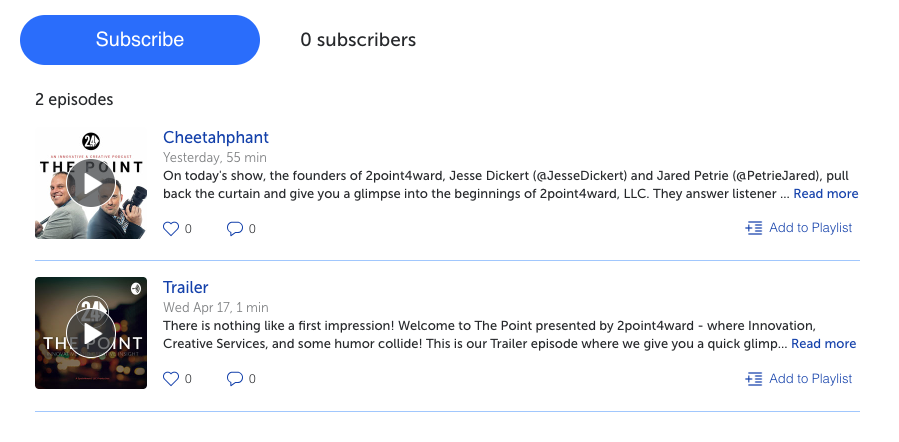This screenshot displays a playlist interface. At the top left corner, there is a prominent blue button labeled "Subscribe" in white text. The user currently has zero subscribers. Two episodes are listed in the playlist. 

The first episode, titled "Cheetah Fart," was uploaded yesterday and has a duration of 55 minutes. The episode features the founders of Two Point Forward, Jesse Descartes (@JesseDescartes) and Jared Petrie (@PetrieJared), who discuss the origins of Two Point Forward LLC and answer listener questions. The episode thumbnail shows two men standing back-to-back, with one holding a camera. A "Read more" link is available for additional details.

The second item is a trailer for the series, uploaded on Wednesday, April 17th, with a runtime of one minute. The trailer introduces the series titled "The Point," presented by Two Point Forward, highlighting themes of innovation, creative services, and humor. It provides a brief overview to entice new listeners, with a "Read more" link for further information. 

Beneath each episode, there is a blue "Add to Playlist" link for user convenience.